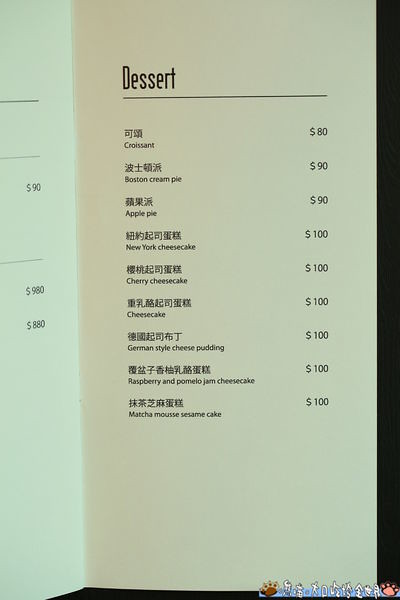The image features a detailed look at a dessert menu, showcasing two pages, with a portion of the preceding page and a complete page fully visible within the frame. At the top of the visible page, the word "Dessert" is prominently written and underlined with a black ruler. The entire menu text is printed in black ink. The layout consists of dessert names listed on the left and their corresponding prices on the right.

The dessert names are initially presented in Chinese characters, numbering nine in total. Each name is followed by its English translation, although the English text is difficult to read in the picture. 

Here are the listed prices for each dessert:
1. $80 
2. $90 
3. $90 
4. $100 
5. $100 
6. $100 
7. $100 
8. $100 
9. Price not visible in the image.

Decorative elements appear at the bottom of the page, including what seem to be dog paw prints and some colorful designs, possibly added digitally.